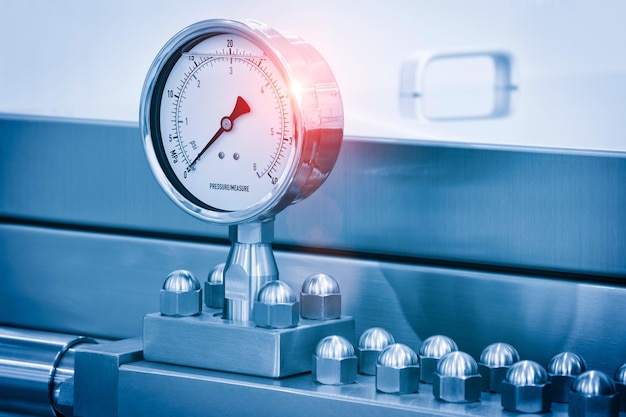The photograph captures a detailed close-up of a pressure gauge mounted on a metallic, square-shaped base. The gauge itself is round with a white face featuring a black semicircle and multiple black notches indicating intervals of 5, from 0 to 40. At the bottom center of the face, the text "pressure measure" is clearly visible. A red needle prominently points to zero. The gauge is encased in a silver, round border, which is connected to a silver knob or cylindrical structure. Surrounding the gauge, the metallic surface and its base are painted in blue. The base is secured with multiple nuts and bolts at the corners, also painted blue, which attach the gauge to a larger piece of metal that shares the same blue hue. Additional nuts and bolts can be seen on the right side and around the base, blending into the blue-painted metallic background.